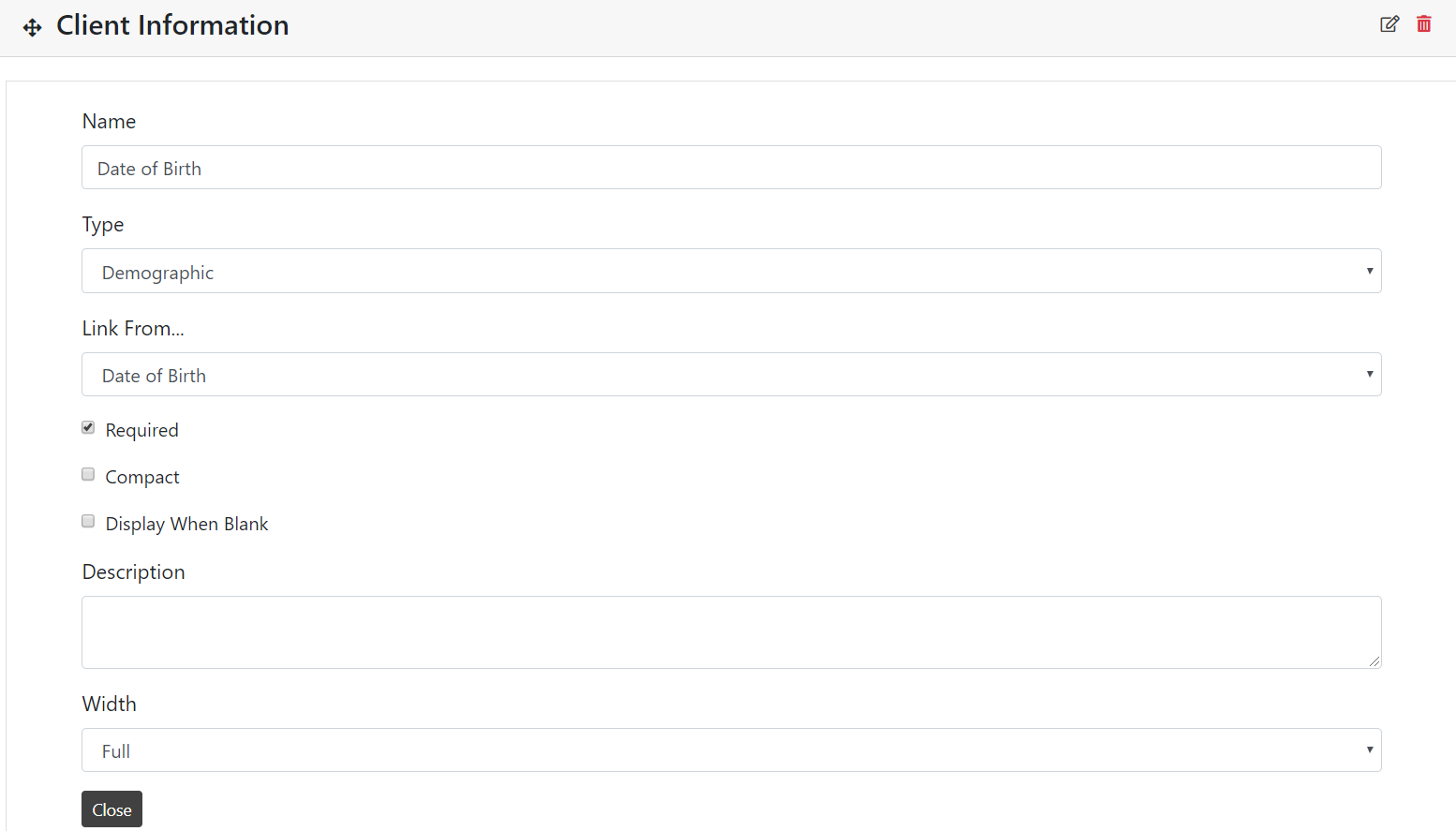The image depicts a web page titled "Client Information" in black text at the top. A black directional sign, resembling a cross with arrows, is prominently displayed. To the right, there's an edit box featuring a pencil icon along with a red trash icon for deleting entries. The form includes fields for "Name" and "Date of Birth," followed by a "Type" field labeled "Demographic." Below the "Date of Birth" section, there's a note that reads, "Link from Date of Birth." Three checkboxes provide additional options: the first, labeled "Required," is checked, while "Compact" and "Display When Blank" remain unchecked. A larger text box, intended for descriptions, is left completely empty. Next to this, a drop-down marked "Width" shows "Full" as the selected option. Finally, at the bottom left corner of the page, there's a black button labeled "Close" in white text. A white outline frames all the fields and elements on the form, adding structure to the layout.